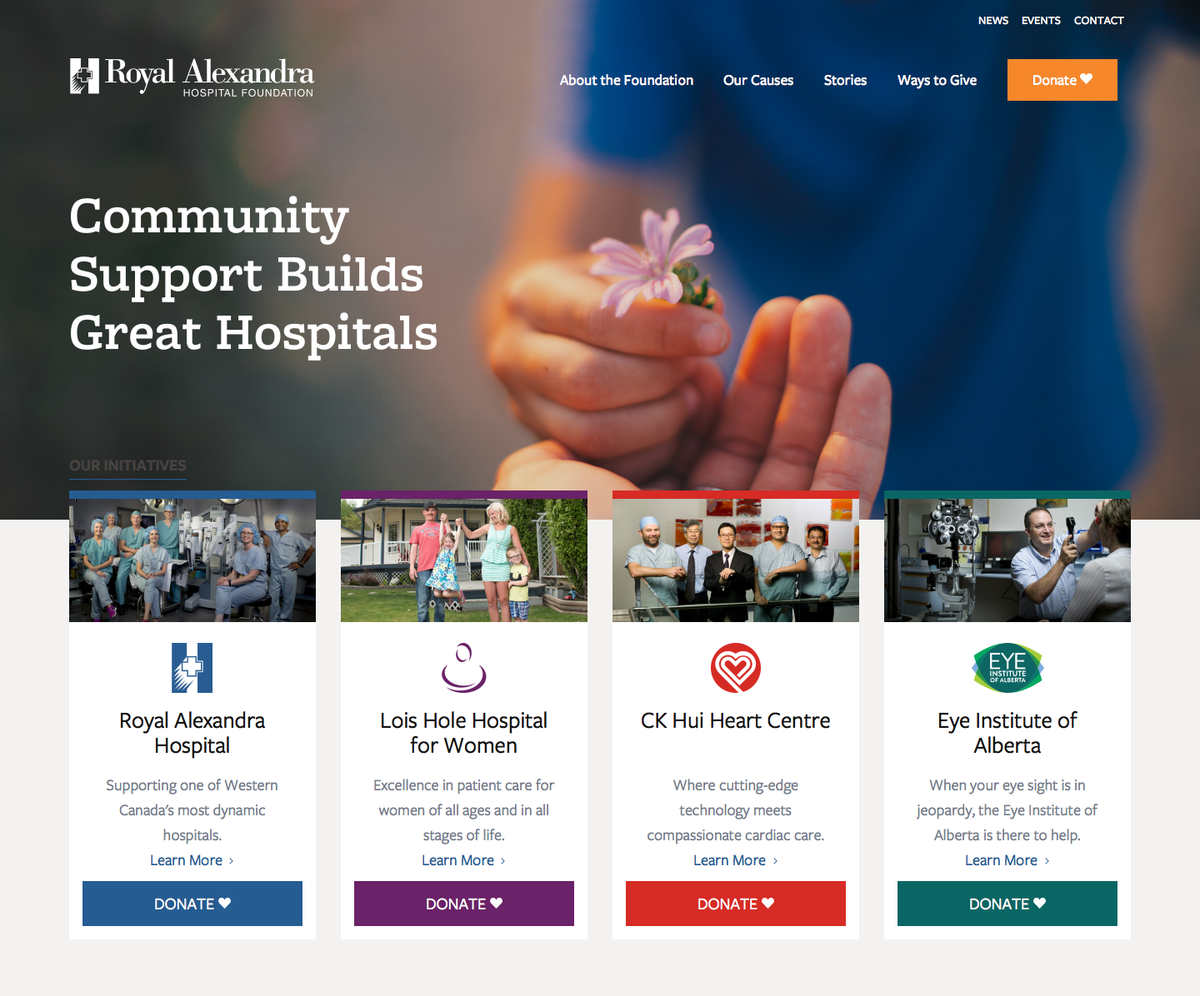The webpage for the Royal Alexandra Hospital Foundation is presented with a professionally designed layout. In the upper left-hand corner, the foundation’s name is prominently displayed in white text. Adjacent to it, a navigation menu offers options such as "About the Foundation," "Our Causes," "Stories," "Ways to Give," "News," "Events," "Contact," and "Donate," all also in white text. The "Donate" option stands out with an orange box around it and a white heart icon beside it.

A central image features an adult and a child holding hands, the child clutching a pink flower seemingly about to present it to the adult. Both individuals are wearing blue shirts. To the right of this image, under the foundation's name, a slogan reads: "Community Support Builds Great Hospitals," also in white text.

Below the main banner, four distinct sections with colored borders present various facets of the foundation's work. 

1. **Royal Alexandra Hospital** (Blue Border):
   - **Image:** Doctors
   - **Description:** "Royal Alexandra Hospital supporting one of Western Canada's most dynamic hospitals."
   - **Call to Action:** "Learn More"
   - **Donate Button:** Blue

2. **Lois Hole Hospital for Women** (Purple Border):
   - **Image:** A family (mom, dad, boy, and girl) interacting warmly, with the parents lifting the daughter.
   - **Description:** "Excellence in Patient Care for Women of All Ages and All Stages of Life."
   - **Call to Action:** "Learn More"
   - **Donate Button:** Purple

3. **CK Hui Heart Centre** (Red Border):
   - **Image:** Doctors and a business person
   - **Description:** "Where Cutting Edge Technology Means Compassionate Cardiac Care."
   - **Call to Action:** "Learn More"
   - **Donate Button:** Red with a red heart icon

4. **Eye Institute of Alberta** (Green Border):
   - **Image:** An eye doctor with a patient
   - **Description:** "When Your Eyesight is in Jeopardy, the Eye Institute of Alberta is There to Help."
   - **Call to Action:** "Learn More"
   - **Donate Button:** Green

Each section emphasizes the hospital's various specializations and services, encouraging visitors to learn more and contribute through clearly marked donation options.